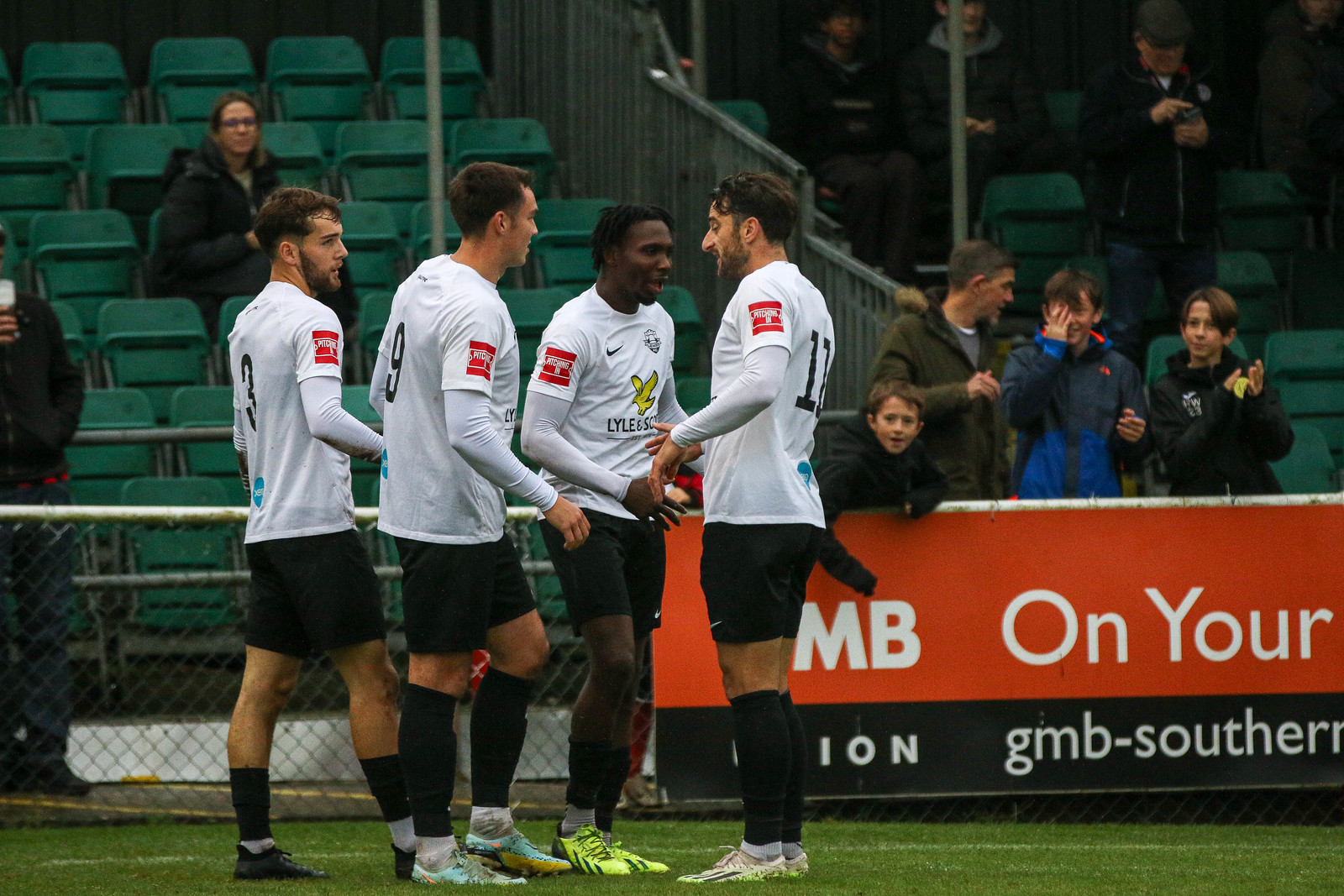The photograph captures an outdoor daytime scene of a soccer game on a grass field. Four players, dressed in white uniforms with black numbers on the back, black shorts, black socks or shin guards, and multicolored cleats, are standing and chatting. Among them, one appears to be African American, while the others are Caucasian or possibly Hispanic. Behind them, there is a metal chain-link fence adorned with advertisements, including a prominent red and black sign reading "MB On Your GMB Southern." A young boy is seen hanging off this sign, watching the players. Beyond the fence, green seats in the stands can be seen, separated by railings into different sections. A few people are seated, including a noticeable woman, while others are standing around, mostly men. The sky appears overcast, suggesting an imminent rain, and many people are wearing jackets, indicating it might be a cold day.